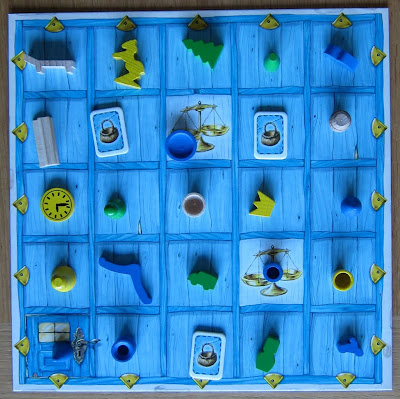The image showcases a square board divided into a 5x5 grid with a total of 25 squares, each filled with a unique or repeating small object. The entire board and its grid lines are painted in various shades of blue, with the objects standing out due to their colorful contrast. The objects, which seem to be crafted from materials such as wood, plastic, or ceramic, include a variety of items: a Christmas tree, multiple clocks, domino-like pieces, cups, pawn-like pieces, and basket illustrations. Notably, there are also items resembling foam shapes, bottle caps of different colors, and a yellow crown. The outer perimeter of the board is adorned with small yellow triangles, with each corner square featuring two triangles and other perimeter squares having one. The scene captures a downward view as if looking overhead at what resembles a blend between a board game and an art piece, leaving its exact purpose ambiguous.